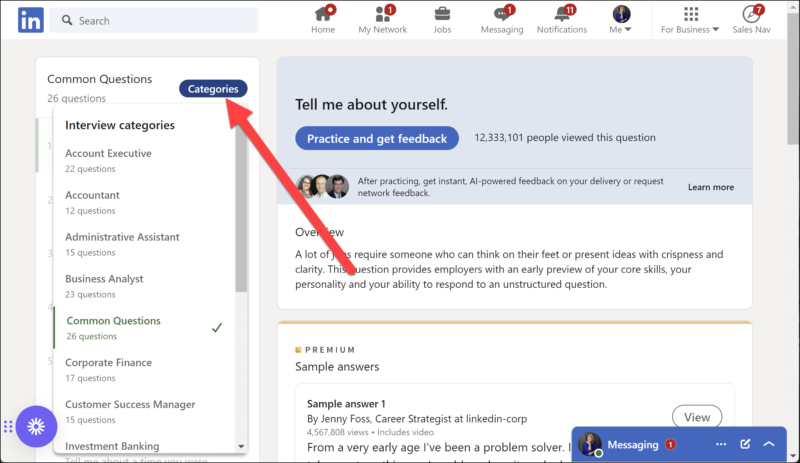The image displays an interface from what appears to be a professional networking platform. In the top left corner, there is a blue box containing the stylized lowercase letters "in." Adjacent to this, a standard search bar sits, followed by navigation options labeled: Home, My Network, Jobs, Messaging, and more.

The primary content starts with a bold heading titled "Common Questions," under which various categorized topics are listed. Below this heading is a vertical scroll bar, indicating the presence of additional interview categories accessible by scrolling down.

To the right, there is a section dedicated to communication, detailing its functionalities. Prominently featured within this section is a labeled area titled "Tell Me About Yourself," which includes both an overview and sample answers for interview preparation.

A large red arrow, angling diagonally, connects the "Overview" text in the "Tell Me About Yourself" section to the "Categories" heading, suggesting a guided flow from understanding general concepts to exploring specific categories.

In the bottom right corner, there is an active messaging section, indicating ongoing conversations. The integration of these elements within the interface suggests a user-friendly guide designed to assist with the navigation and preparation for interview scenarios.